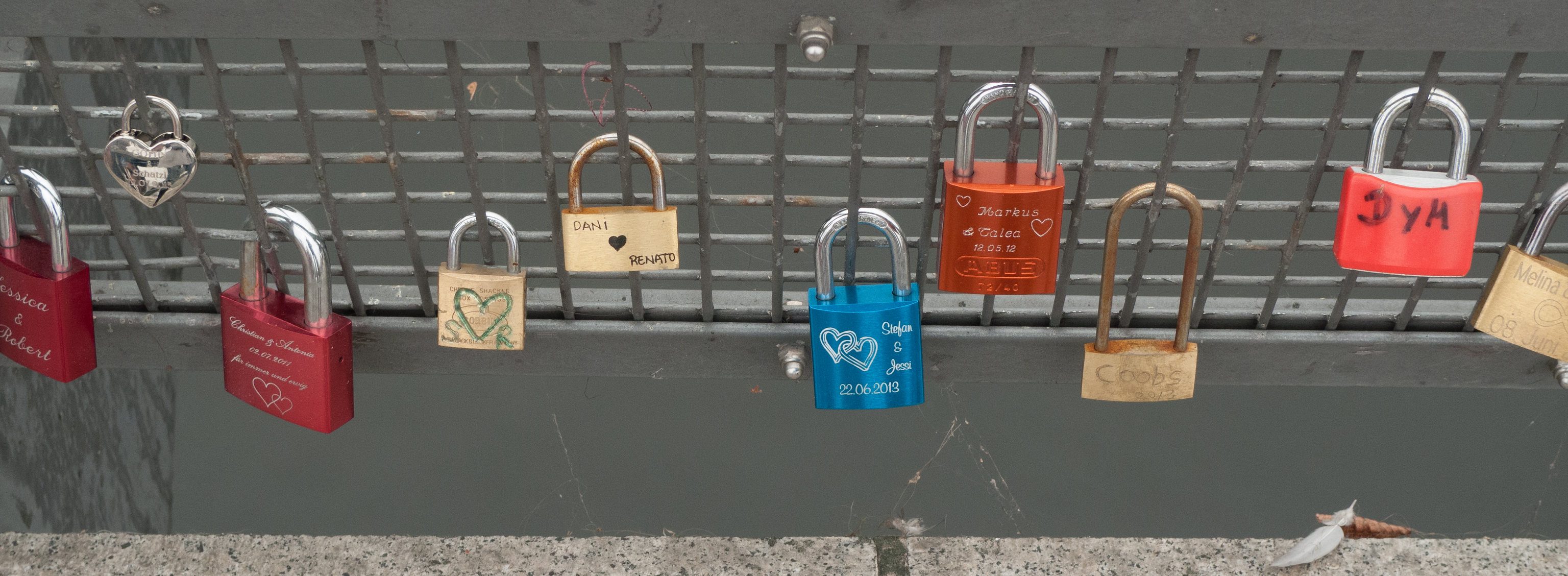In this photo, the central focus is a collection of vibrant padlocks fastened to a metal grate set against a gray background. The assortment of padlocks—numbering around ten—includes various colors: three red, one bright pink, one blue, one silver, and four gold. Some of the locks bear engraved or written names and initials, such as "Jessica and Robert," "S and R" with a heart, "Danny with a heart and Renato," "Stefan and Jesse 2206-2013," "Koobs 13," "Marcus and Caleb with a heart 1205-12," "Sia or DyM," and "Melina OB June." These padlocks, often symbols of love or memorable visits, are securely attached to the metal structure, which may be part of a bridge or another type of fence or grate. Below them, at the bottom of the image, a concrete block is visible alongside what appears to be a bird's feather in the lower right-hand corner, adding a touch of natural element to the scene.